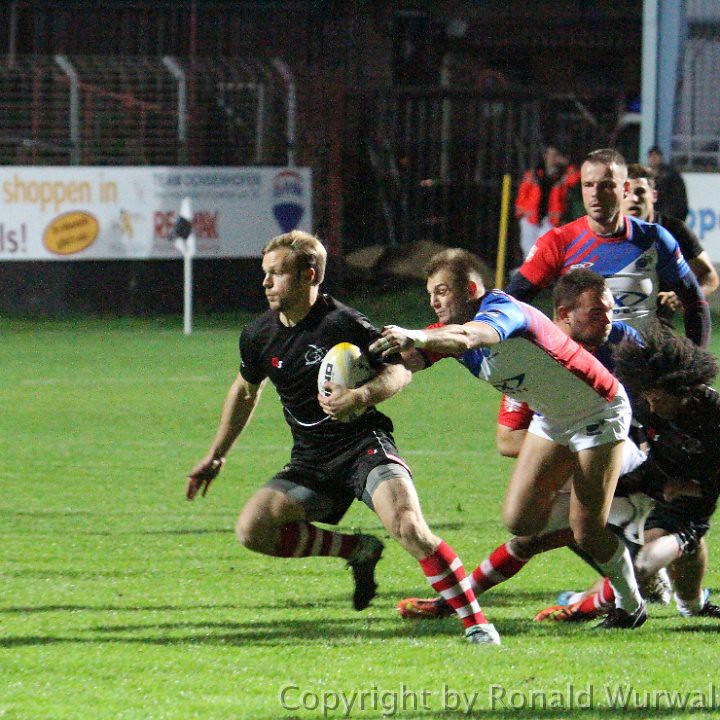The image captures an intense moment of a nighttime rugby match on a lush, green turf field. Central to the image, slightly to the right, are four to five rugby players in motion. The key player, wearing a black shirt, black shorts, and distinctive red and white striped socks, is running with the rugby ball. A determined opponent in a vibrant red, blue, and white jersey, paired with white shorts and socks, lunges at him in an attempted tackle. Three to four other players trail behind them, moving in the same direction, likely trying to support or intercept. The background is dotted with banners, sponsor signs, and a fence enclosing the arena. Towards the bottom right corner, a watermark reads "Copyright by Ronald Warwall." Additional details include empty audience benches to the left and a coach in a red coat observing the action. The setting is clearly outdoors, illuminated by night lighting, adding to the dynamic atmosphere of the ongoing game.